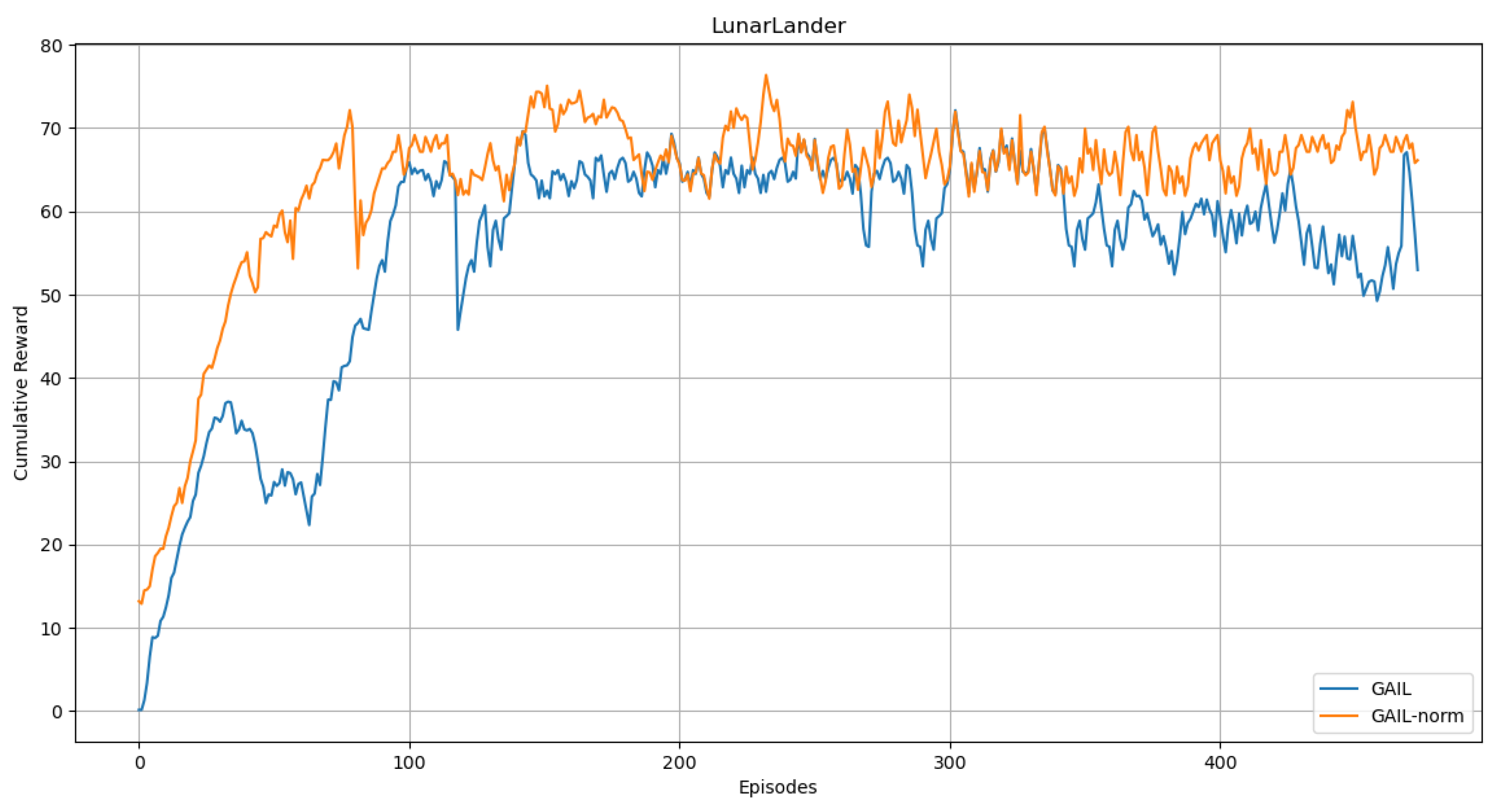The image features a detailed graph with a black background on the sides and a gray rectangle across the top. The vertical axis on the left side ranges from 0 to 80 in 10-unit increments, while the horizontal axis spans from 0 to 400, marked in 100-unit increments (100, 200, 300, 400). The graph is divided into five sections, each marked with lines corresponding to the vertical axis values. Two distinct lines traverse the graph: an orange line labeled "Gale Norm" and a blue line labeled "Gale." 

The orange line, starting around the value of 14, ascends steadily across the entire graph to a peak of approximately 70. The blue line, in contrast, begins at 0 and displays a zigzag pattern with fluctuations, peaking at about 67. 

The graph's title at the top reads "Lunar Lander Cumulative Reward." At the bottom, there is a legend enclosed in a gray-bordered square explaining the color coding of the lines: "Gale" corresponds to the blue line, and "Gale Norm" to the orange line. The colors used in the graph include black, white, gray, orange, and blue. The graph appears to represent some kind of measurements, possibly related to sound waves or lunar lander performance data.